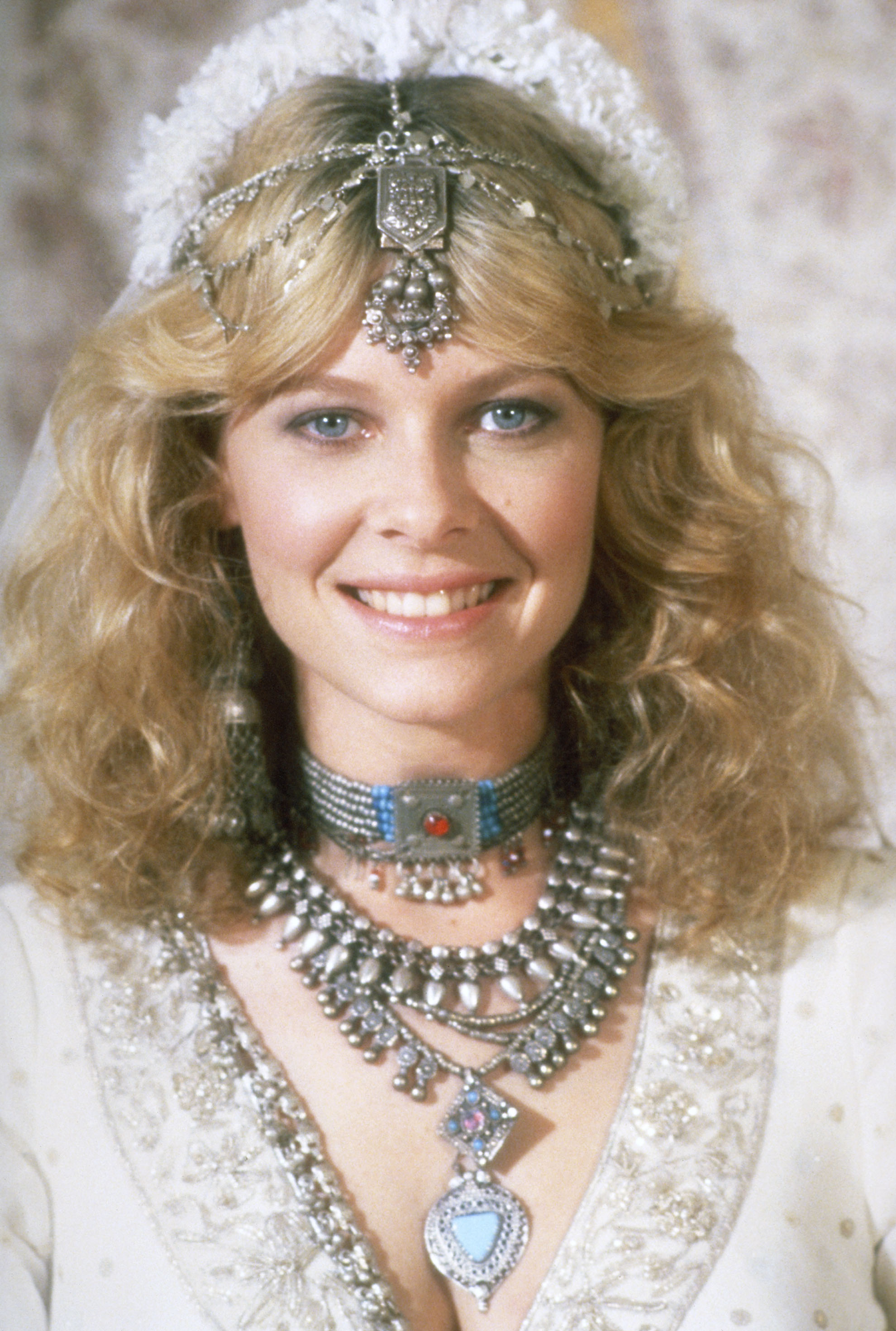The image features a young, blonde woman with long, curly hair cascading down either side of her face. She is positioned directly in the center of what appears to be a formal setting. The background is elegantly blurred, lending a professional, almost ethereal quality to the photograph. The woman's attire is strikingly ornate, reminiscent of a wedding dress, predominantly white and low-cut, revealing a subtle hint of cleavage.

Her ensemble is adorned with an abundance of jewelry. She wears large, dangling earrings and a tightly-fitted choker made of beads, accented with a central red jewel set in a square silver frame. Beneath the choker rests another elaborate silver necklace embellished with stones and featuring a blue gemstone. Layered over it all is an intricate metallic headdress that doubles as a veil, complete with a bouquet-like arrangement or veil train on top. The headdress extends down to her forehead, where it is adorned with a piece of jewelry featuring four chains and an elaborate pendant.

The woman’s blue eyes, accented by her friendly smile, convey a sense of warmth and grace. The colors in the image include a harmonious palette of white, silver, light blue, blue, red, pink, brown, yellow, and grey, enhancing the overall opulent appearance of her outfit and accessories.